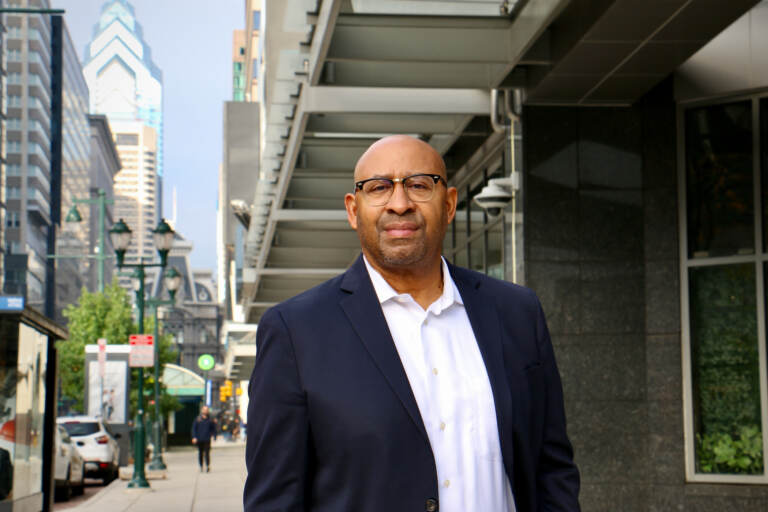In this image, a heavyset Black man is posing for a photo in a bustling urban area. He stands on a gray sidewalk in front of a black building with a white metal canopy and windows running along its side. The man is dressed in a navy blue suit coat over a white buttoned-up collared shirt, with the coat left unbuttoned. He wears a pair of black glasses with wire frames below and a gold trim bar between the lenses. Sporting a slight beard and a clean-shaven bald head, the man exudes a subtle, closed-mouth smile. In the background, two white cars are parked by the curb on the left, and a green lamppost with two lamps stands nearby. Further back, a towering building with three triangular shapes at the top rises against a bright blue, sunny sky. Another person is visible walking towards the man on the pavement.